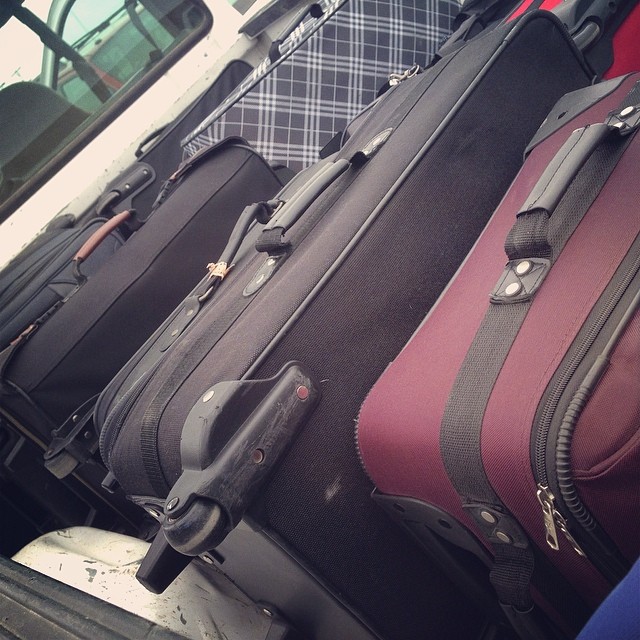The photograph depicts the back of a white truck loaded with a diverse collection of suitcases. The upper left-hand corner reveals the rear window of the truck with black trim, adding context to the scene. The truck's open door and part of the front seat are visible on the right side. In the truck bed, eight suitcases of various colors, designs, and sizes are closely packed together in two rows. Notably, three black suitcases, a maroon one, and a black and light blue checkered one are among the collection. All the suitcases are zippered shut, upright with handles on top, and some have rolling wheels. The cases are described as primarily canvas material, mixing soft-sided and hard-sided types. The organized arrangement suggests the suitcases are being transported, likely towards a luggage carousel.